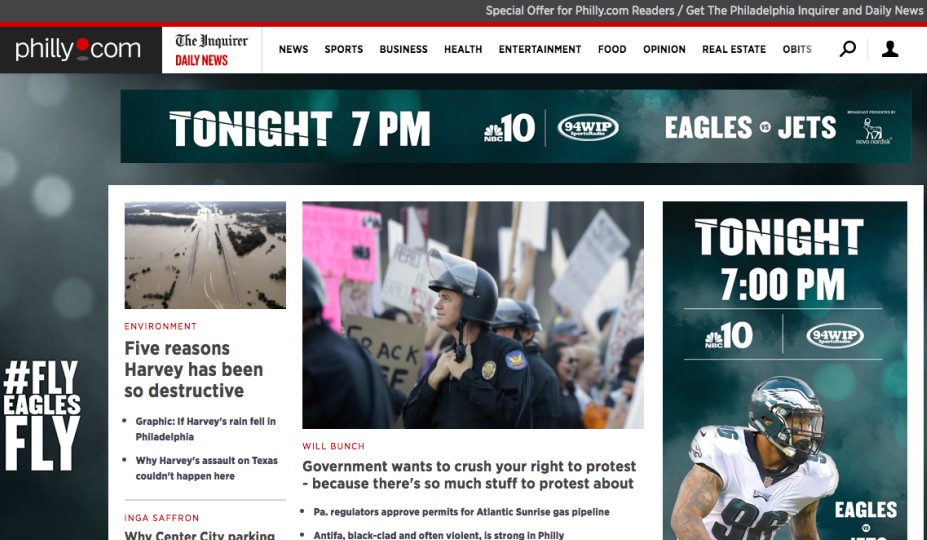This is a cropped screenshot of the philly.com homepage. In the top left corner, the philly.com logo is prominently displayed, featuring a distinctive black dot replacing the usual "dot" and a red dot for the letter "i", which adds a unique flair. To the right of the logo, there's a horizontal menu listing various categories: The Inquirer, Daily News, News, Sports, Business, Health, Entertainment, Food, Opinion, Real Estate, and Obituaries. This menu is scrollable to reveal more categories.

On the far right of the menu bar, there is a magnifying glass icon indicating the search function, which expands into a search bar upon clicking. Next to the search icon, there is an account icon.

Beneath the menu, a large banner stretches across the top of the page, advertising an upcoming event: "Tonight 7 PM NBC10, Eagles vs Jets," accompanied by a circular sponsor logo to its left. Articles populate the central portion of the webpage. 

On the far right side, another prominent banner reiterates, "Tonight 7 PM ABC10, Eagles vs Jets." At the bottom left of the image, there is a large hashtag, #FlyEaglesFly, emphasizing support for the Eagles.